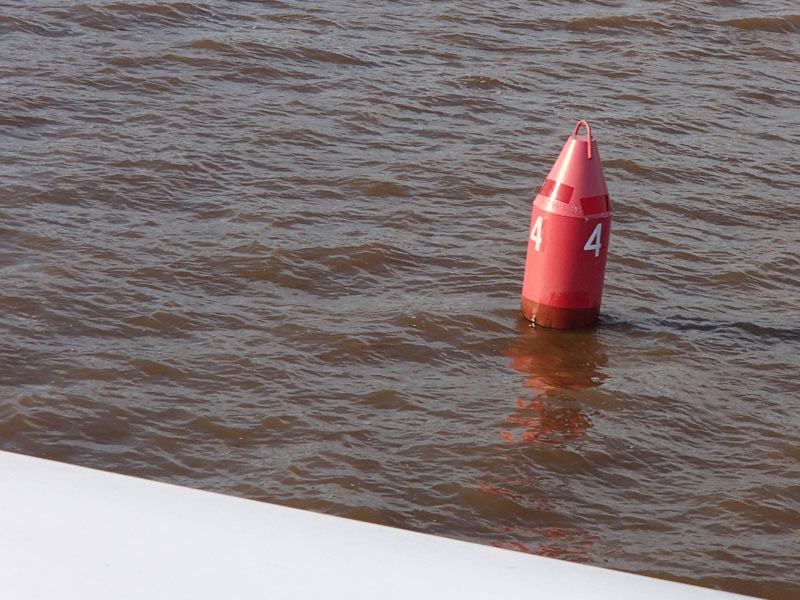The photograph captures a red buoy floating in a murky, brown body of water. The buoy displays the number "4" twice in white text. The buoy's top is a brightly colored cone, with varying shades of red and pink, and features a thin metal bracket that resembles an upside-down horseshoe at its peak. Towards the bottom, which sits in the water, the buoy appears dirtied with mud, giving it a brownish hue. The water itself has waves and ripples, adding texture to the scene. In the foreground, a white rectangular surface, possibly part of a marina, jetty, or a boat, is visible. The water casts reflections of the buoy, with red hues dancing on its surface, accentuating the buoy's presence. A black shadow extends from the back of the buoy, suggesting it is sticking out of the shallow water.